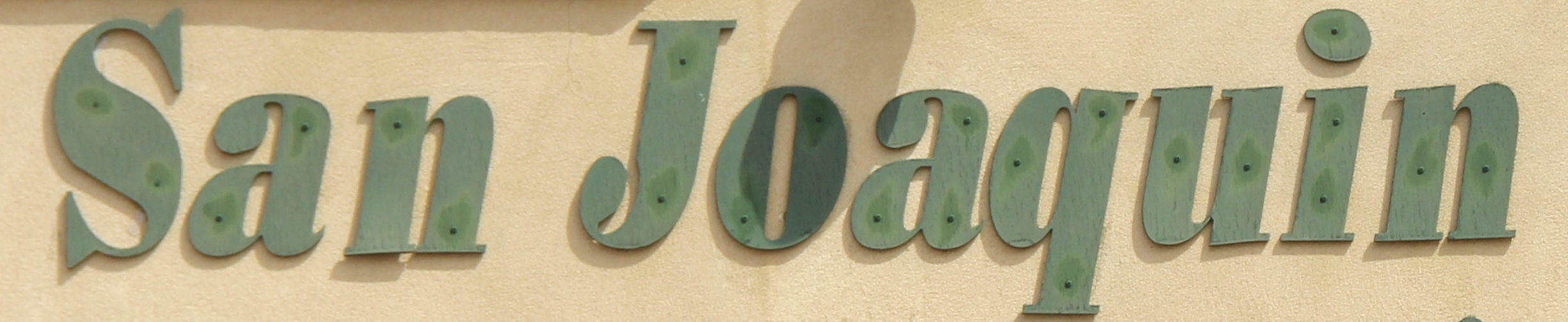The image features a sign that appears to be mounted on the exterior wall of a storefront or restaurant. The wall is primarily a tan color with a subtle orange hue, creating a very bright and inviting background. The sign itself consists of green lettering that spells out "San Joaquin." The text is displayed in a distinctive font where the capital 'S' in "San" has a wide middle section, giving it a dynamic thick-to-thin shading effect. The lowercase 'a' and 'n' in "San" and the entire word "Joaquin" are in the same font style, making the sign both aesthetically pleasing and easy to read.